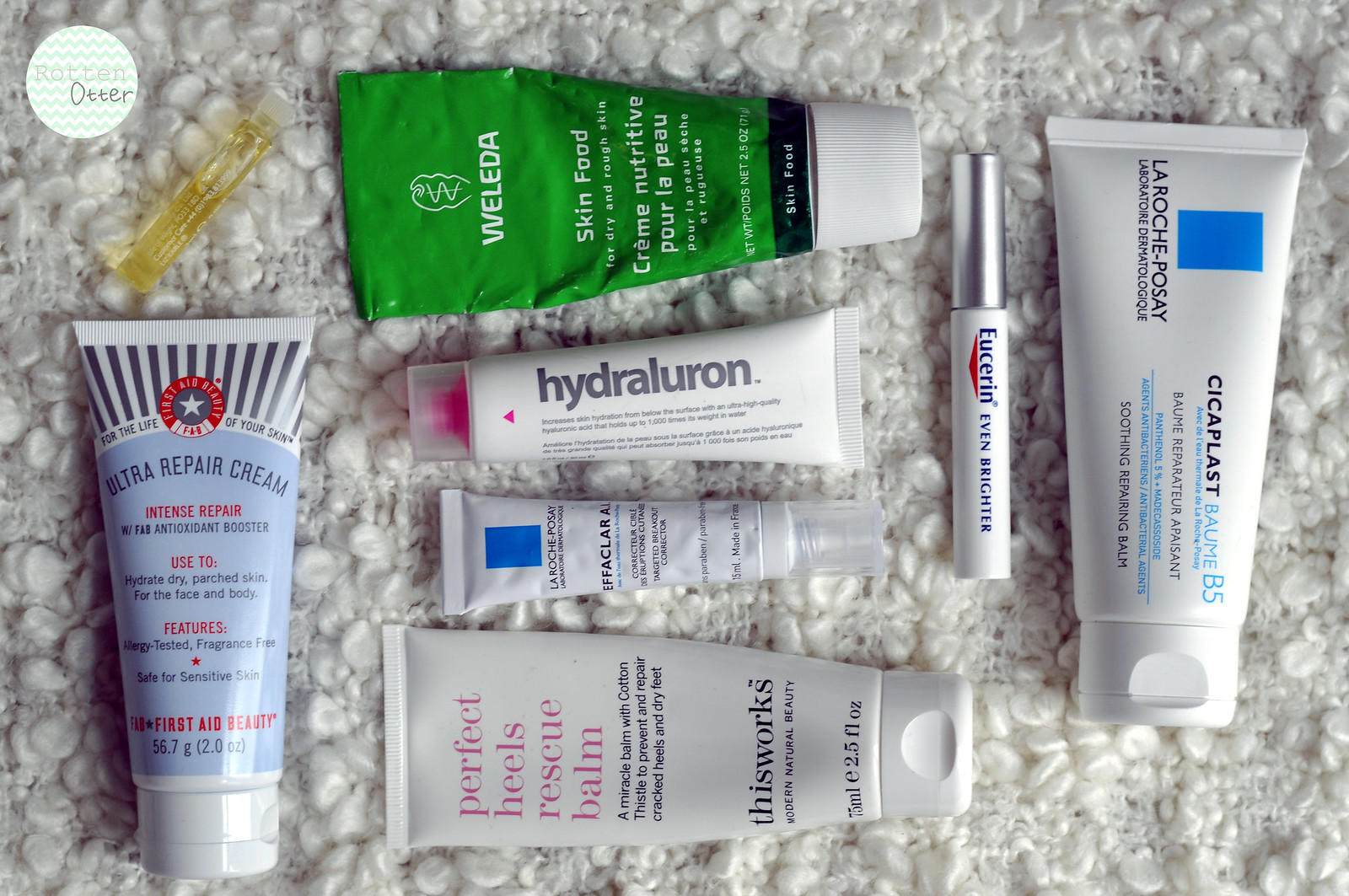The image captures a collection of eight skincare and hygiene products neatly arranged on a textured surface, which appears to be either a bath rug or the top of an overnight bag. Positioned in the upper left corner is a circular logo bearing the name "Rotten Otter."

The assortment includes the following items:
1. A perfume sample.
2. An Ultra Repair Cream.
3. Weleda Skin Food.
4. A bottle labeled "Hydraluron," suggesting it is a lotion or serum.
5. A small tube of La Roche-Posay product, possibly a skin cream.
6. A Perfect Heels Rescue Balm.
7. A Eucerin Even Brighter tube, which resembles a mascara applicator.
8. Another La Roche-Posay product, Cicloplast Balm B5, and a tube marked "Effaclar AI."

Each item is distinct in its packaging and intended use, representing a well-rounded selection of skincare essentials.